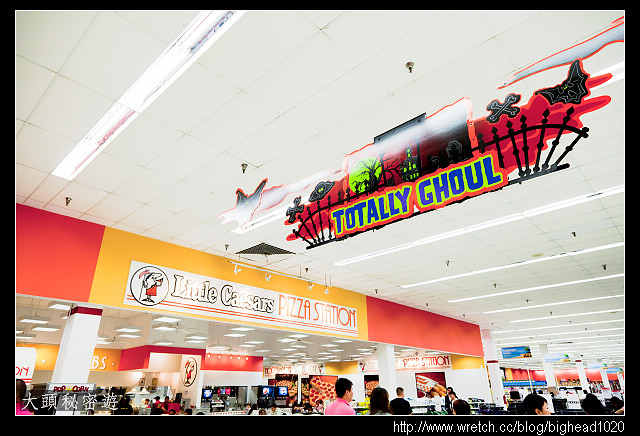This photograph depicts an interior scene of what appears to be a store, quite possibly located within a mall setting in Shrem, China, as suggested by the presence of Chinese characters in the bottom left-hand corner. Dominating the upper section of the image, the white tiled ceiling is lined with rows of rectangular strip lights. Centrally hanging from the ceiling, a Halloween-themed sign with a lime green background and blue "Totally Ghoul" text features a haunted house, black fence, and a black bat artwork. Beneath this festive decor, an orange and yellow banner advertises a "Little Caesars Pizza Station," with the Little Caesars logo prominently displayed.

In the middle ground, there is a visible row of soda machines accompanied by a noticeable popcorn machine, enhancing the food-centric ambiance of the area. Off to the right, additional signage highlights further offerings from Little Caesars. Below the bustling scene filled with patrons, presumably waiting to order or seated at tables, employees in recognizable uniforms attend to the busy station. The black border and a small webpage URL in white text in the bottom right corner, alongside detailed images of pizzas and other snacks, add to the detailed depiction of this lively, pizza-themed service area.